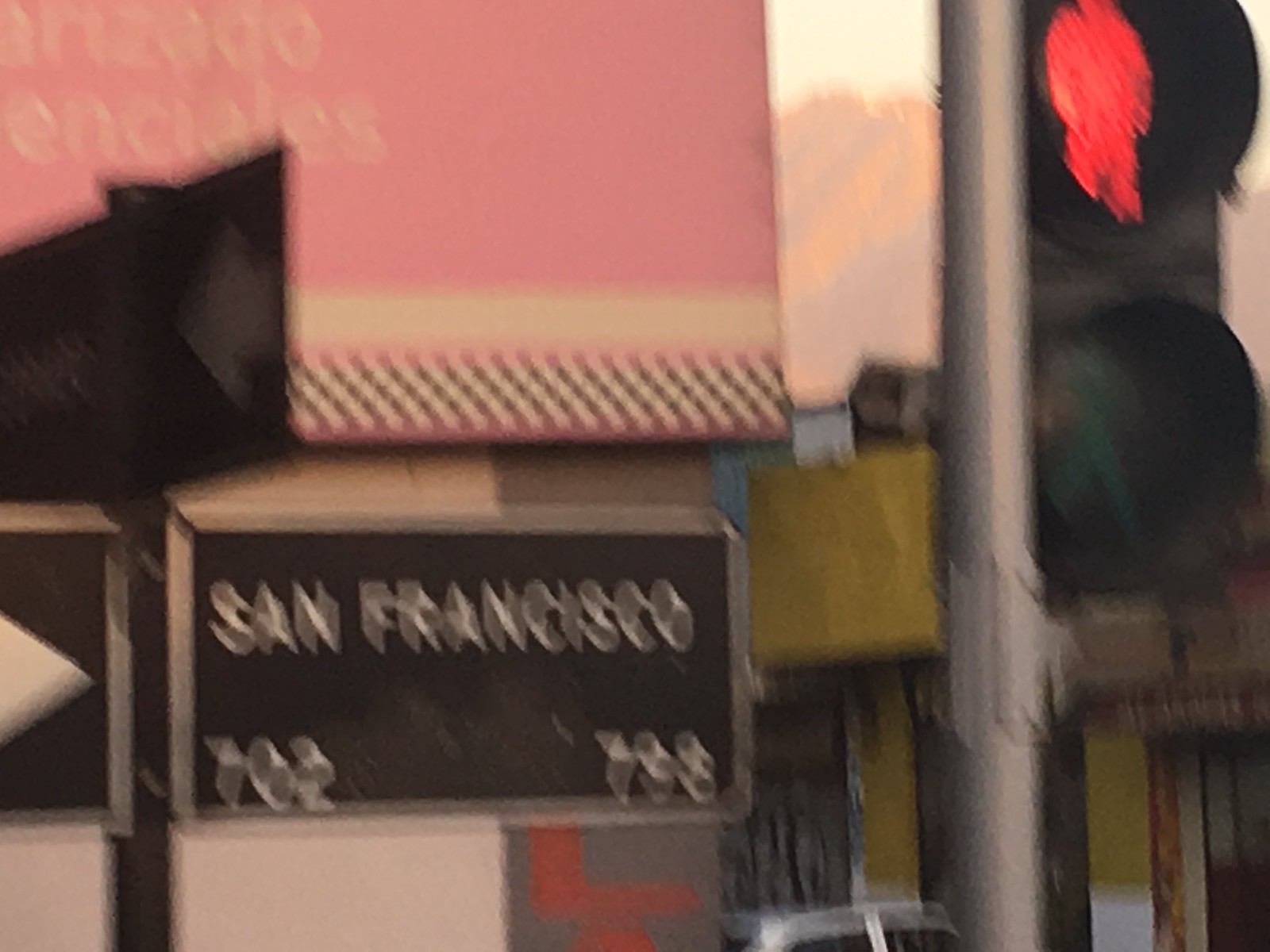This photograph features an urban street scene dominated by a "Walk Don't Walk" sign affixed to a metal pole on the left side of the image. The "Don't Walk" indicator is illuminated in red. On the opposite side, several street signs are visible, though one is notably blurry. It reads “San Francisco” with additional numbers beneath it, rendered in white font against a black background. 

In the background, there's a grayish-white building adorned with a striking red stripe. Adjacent to it is another structure with olive green accents. Atop the gray and white building, there is a conspicuous pink and white sign that includes a distinctive black and white checkered pattern at the bottom, and white text—though the specific words are not discernible. The overall composition captures a vibrant slice of city life, marked by a mix of colors and architectural details.